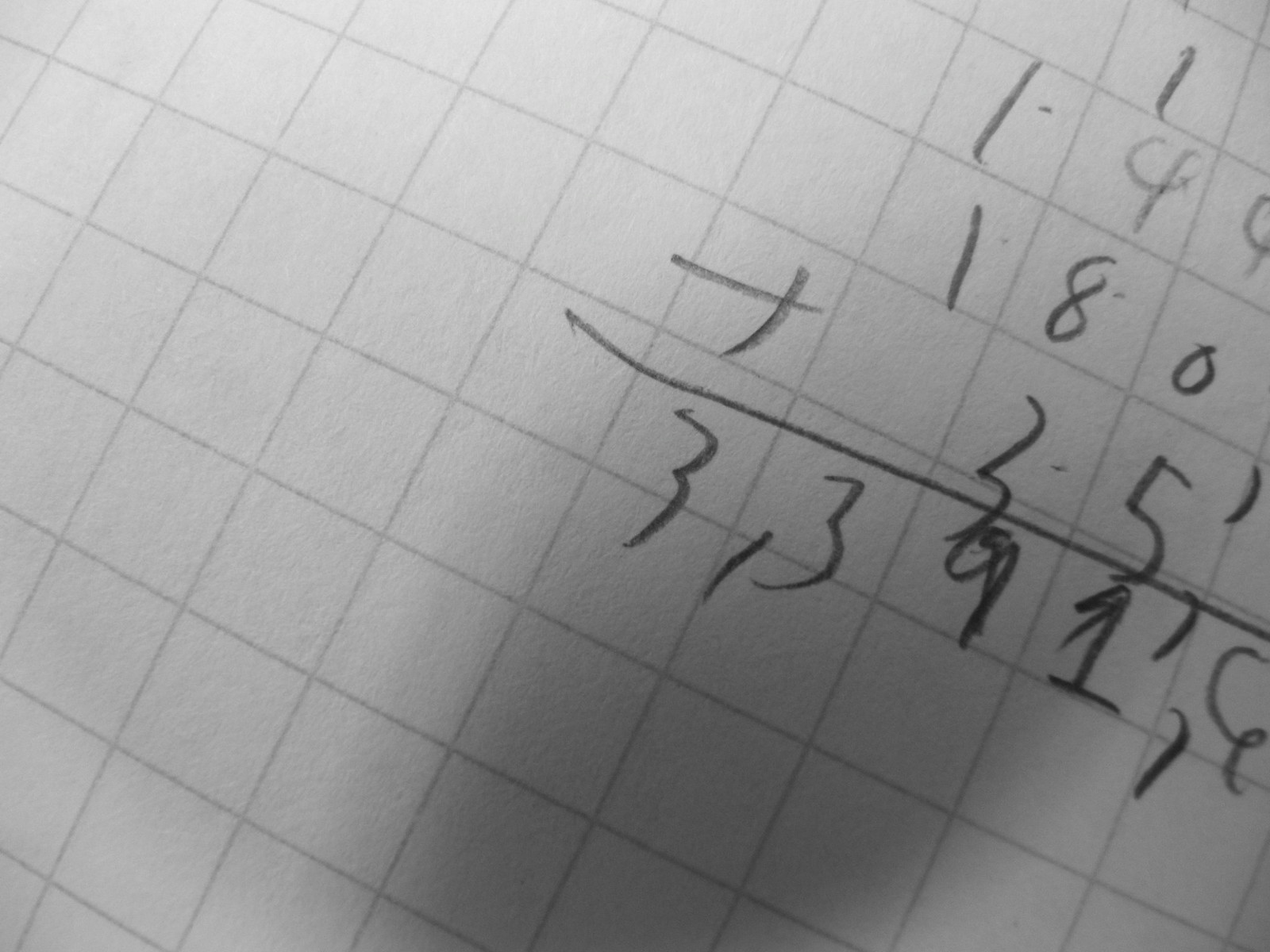The photograph showcases a sheet of white grid paper featuring a series of small black squares arranged in a precise grid pattern. The paper serves as the backdrop for a handwritten mathematical calculation, executed with a graphite or lead pencil. On the right side of the image, partially obscured by a shadow, a sequence of numbers is faintly visible, forming what appears to be an addition equation. The handwritten digits are somewhat messy and difficult to decipher clearly.

The equation starts with a top row of numbers that could be interpreted as either "149," "199," or "144." The second row displays "180," with the '8' distinctly drawn without connecting at the top and the '0' appearing unusually small with overlapping edges. A roughly sketched plus sign (+) is visible to the left of the third row.

The calculated result, partially cut off, seems to be "33916." A dark shadow looms over the right side of the paper, casting the numbers into partial obscurity, while the left side of the paper is illuminated brightly, highlighting the contrast between light and shadow. Despite the shadow, the handwritten numbers remain visible, although challenging to read due to their disordered, scribbling appearance.